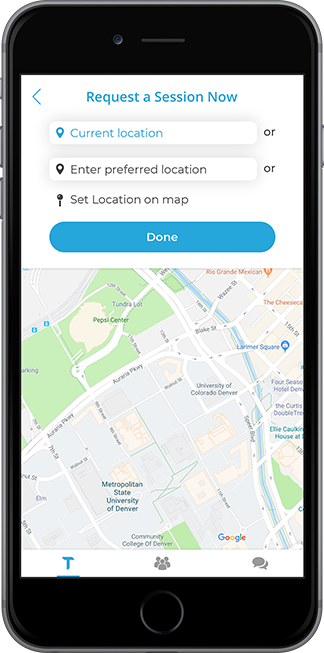A screenshot displayed on a tablet with a black border showcases a Google Maps interface. At the top left, there is a blue less-than symbol beside the text "Request a session now." Below this, a blue location pin icon is labeled "Current location," followed by a black location pin icon labeled "Enter preferred location." Further down, another option titled "Set location on map" appears. A blue "Done" button is positioned beneath these three options.

The Google Maps image itself is extremely blurry, rendering most details unreadable except for the word "university." The map displays a collection of streets, parks, and what appears to be a river. At the bottom of the screen, there are three icons: a blue 'T' shaped icon, an icon representing a group of three people, and an indistinct, gray blur.

This detailed setup indicates an interactive interface for determining and setting a location, though the blurriness of the map complicates its practical use.